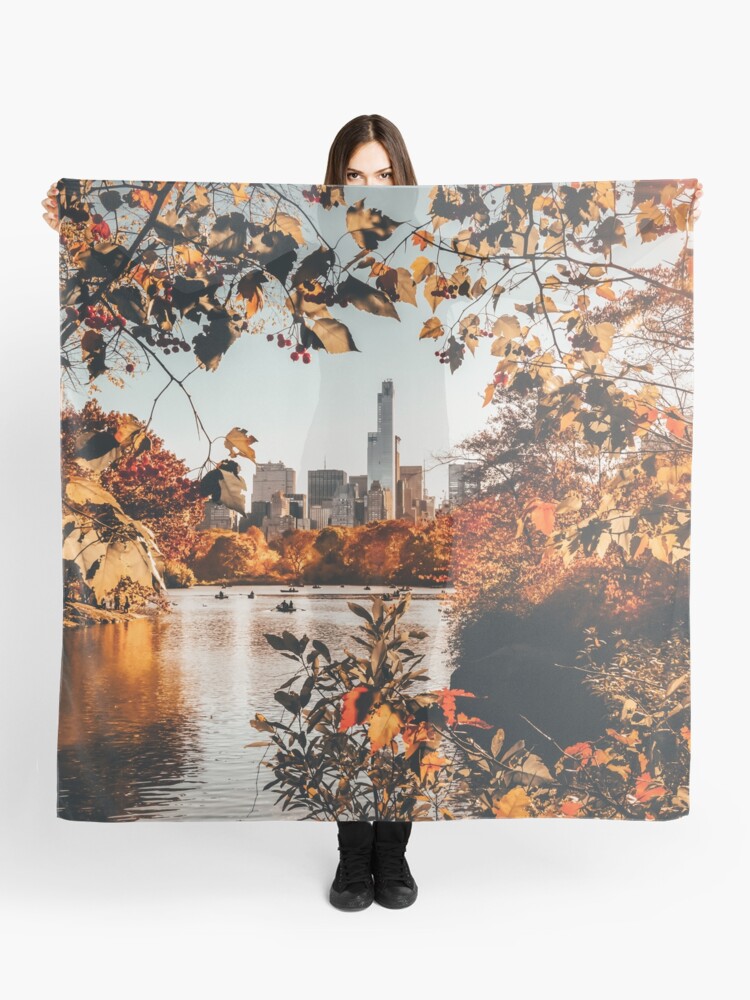In this image, a woman with straight brown hair, dressed in black pants and black shoes, is holding a large tapestry or fabric wall hanging, measuring approximately four feet by four feet. She extends her arms fully, gripping each corner at the top of the tapestry, revealing only her eyes above and her feet below it. The tapestry depicts an autumn scene in Central Park, New York City, characterized by dark, vibrant fall foliage in hues of yellow, brown, and red in the foreground. Just beyond the leaves, a lake with small boats and more autumn-colored trees and bushes can be seen. In the distance, the city's skyscrapers rise against the skyline, completing the picturesque setting.